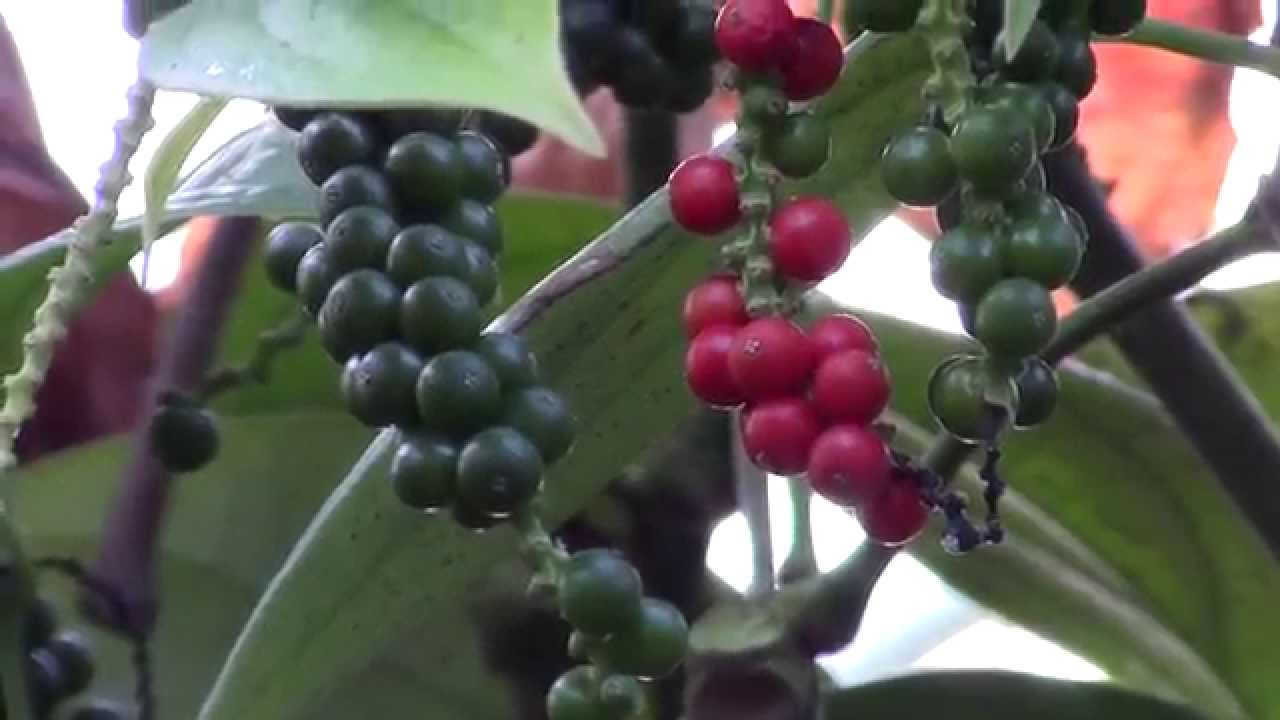A close-up photograph of a plant, though blurry and of low quality, showcases its long, slender green leaves. The plant is adorned with several clusters of small, round seed-like berries. One cluster exhibits a deep, black hue, another a vibrant ruby red, and yet another an olive green. The berries, similar in appearance to peppercorns, appear firm despite their tiny size.